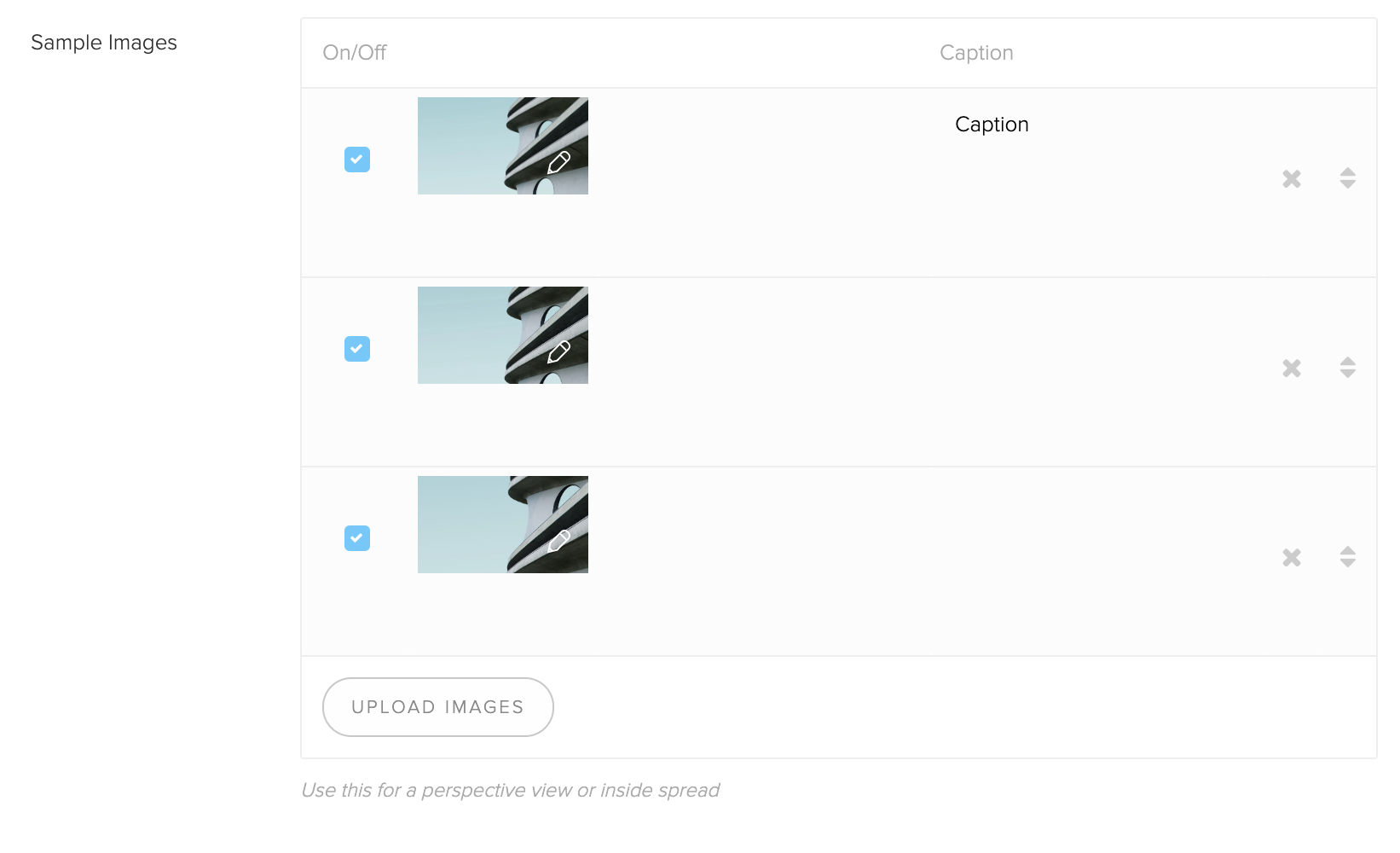The image depicts a user interface with a box that has a light gray border. Outside the box on the left, in black text, it says "Simple Images." Inside the border, there is a thin white header area at the top. On the left side of this header, it reads "On/Off," while on the right side, it says "Caption."

Below the header, there are three light gray-colored rectangles, each containing a blue checkbox marked with a check. Adjacent to each checkbox on the right, there is an image showing the exterior of a building featuring a window against a gray sky backdrop.

In the first rectangle, under a column labeled "Caption," there is text, while the other two rectangles do not have any text under the same column. To the right of each rectangle, there are icons for deletion (X) and reordering (up and down arrows). At the bottom of these sections, there is a button labeled "Upload Images."